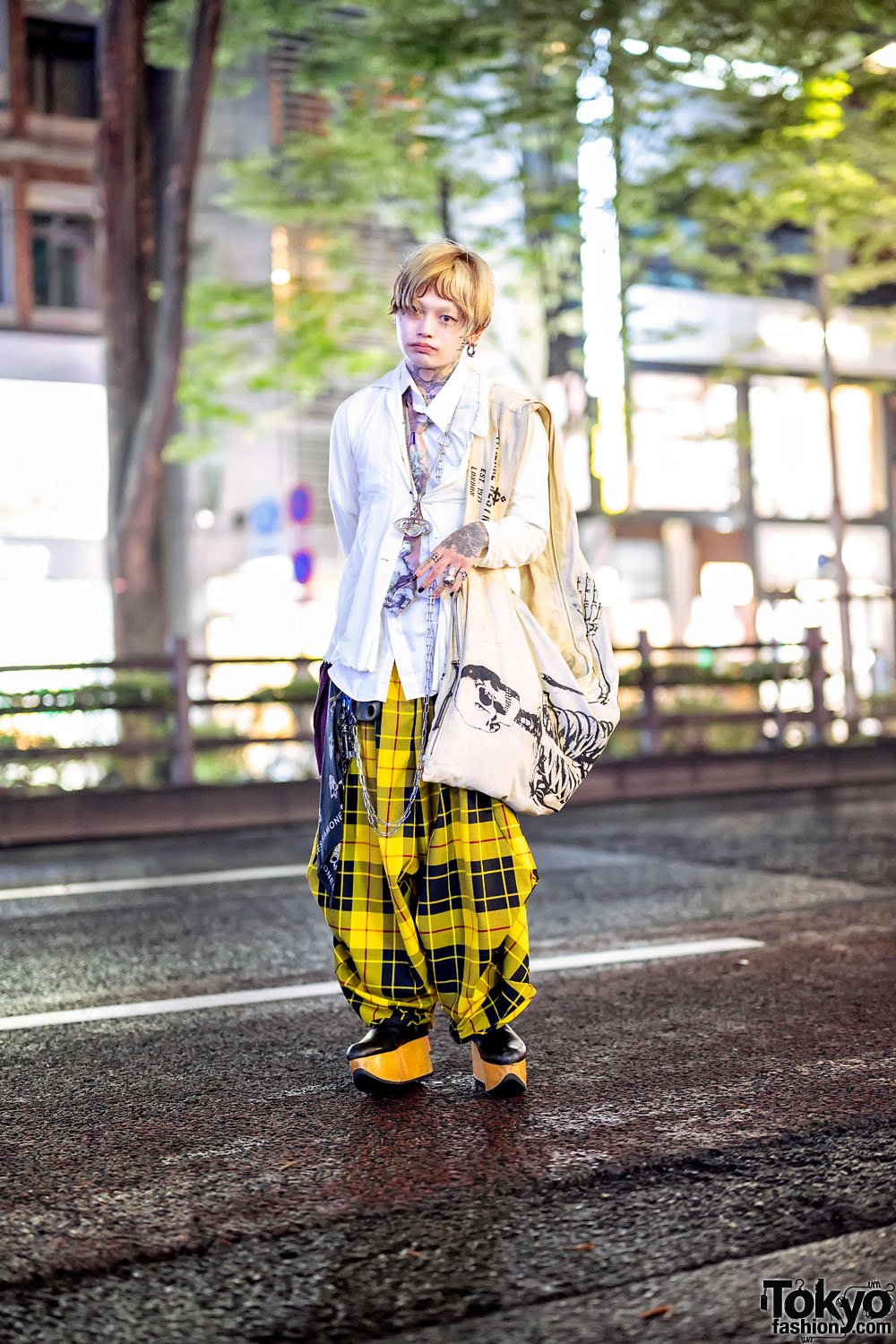The image is an outdoor advertisement showcasing an eclectic fashion outfit. The setting features a street made of rusty pavement in front of a white building with brown window panes. In the background, there is a thin tree with bifurcating branches adorned with greenery, and a low wooden fence lines the street. 

The focal point is a girl wearing yellow and black plaid balloon-type pants, which have a wide-leg style tight at the ankles, reminiscent of clown pants. She pairs these with black platform shoes that have raised yellow soles. Her upper body is dressed in two white shirts, one of which is an oversized bohemian style with long sleeves that hang down to her upper thigh, complemented by a multi-colored pastel tie. Over her left shoulder, she carries a large off-white canvas tote bag featuring a black skeleton design. 

Accessories include a large pendant necklace and several rings on her forefinger, ring finger, and pinky finger. Visible tattoos decorate her left hand, neck, and one side of her face. She has short blonde hair streaked with orange and a hoop earring in her left ear. Her features suggest she might be of Asian descent. The bottom of the image prominently displays the text "tokyofashion.com."